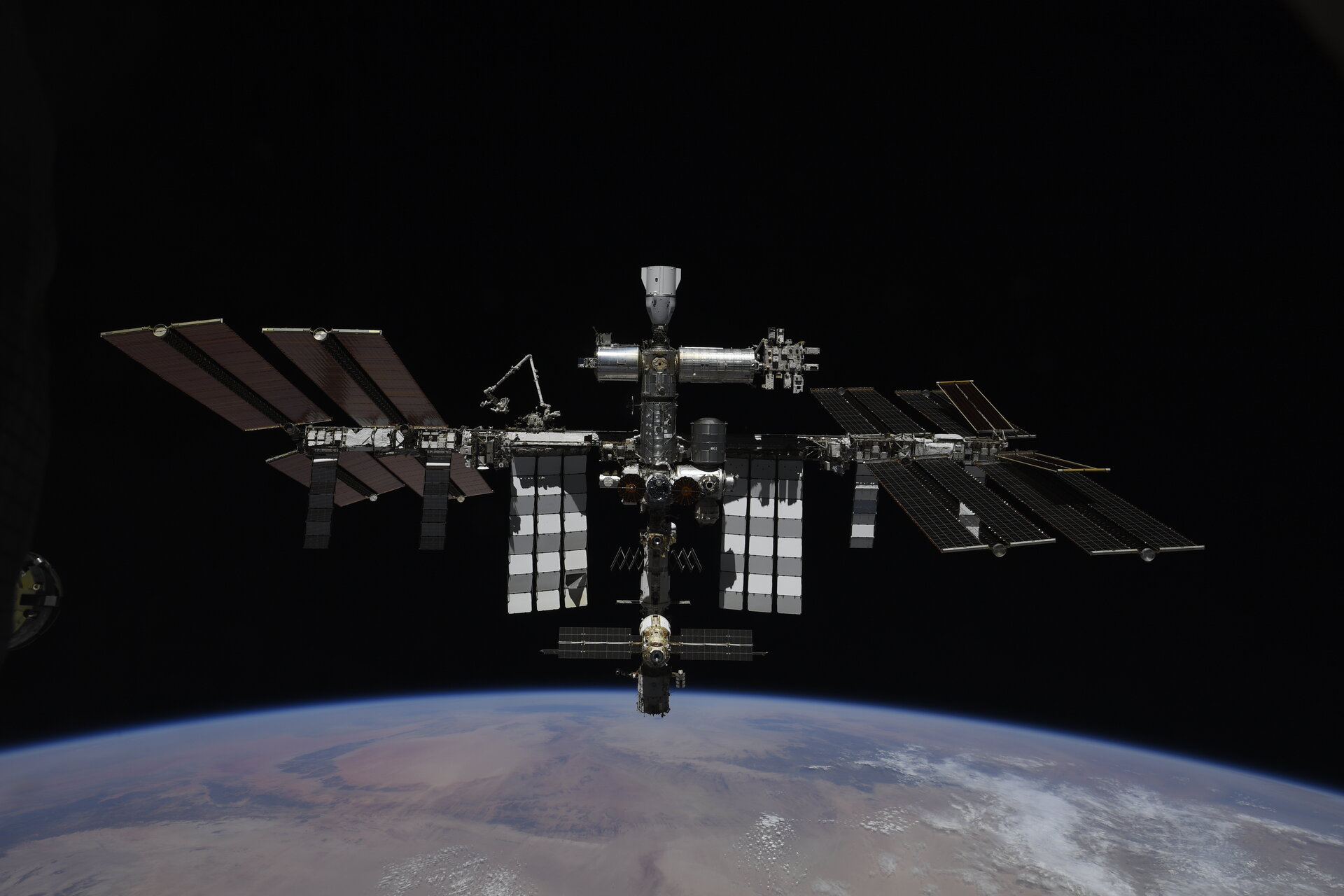The photograph captures an orbiting space station set against the pitch-black backdrop of space, with the Earth's curved surface occupying the bottom quarter of the image. Dominating the center, the station is flanked by extensive solar panels on either side, gleaming with reflections and casting shadows. On the left-hand side, an articulating arm extends over the structure, suggesting the station's sizable scale. The Earth's visible portion shows the ocean and varying weather patterns, including white areas indicative of cold weather and a reddish tinge in one corner. The station, made primarily of silver metals with dark brown panels, appears to be an unmanned satellite designed for data collection or signal transmission, emphasizing technology's role in space exploration.